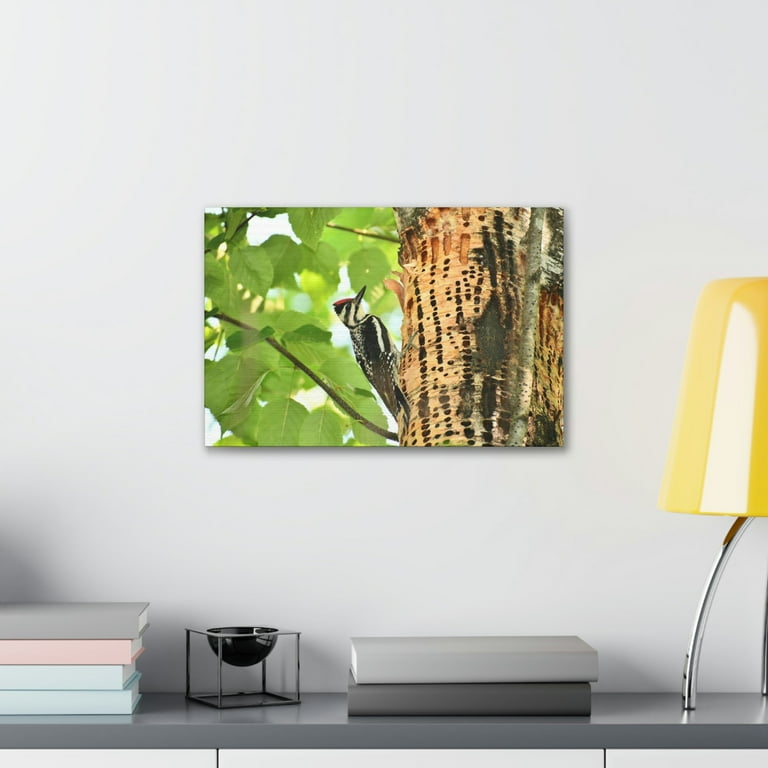This color photograph captures the interior of a sleek and minimalistic office or home office. The focal point is a striking frameless photograph on a white wall, depicting a red-headed woodpecker perched on an orange tree trunk adorned with intersecting black stripes. Green and yellow leaves form the lush background of the bird's scene. On the glossy gray marble countertop below, there are several items meticulously arranged. To the left, a stack of three books rests beside a small piece of art. In the center, two gray books of varying shades are stacked on top of each other, accompanied by a black half-circle candle holder with wax in the center. On the right side of the countertop stands an eye-catching yellow lamp with a silver stem and a yellow and white shade. The clean and organized setup creates a modern and visually appealing workspace atmosphere.